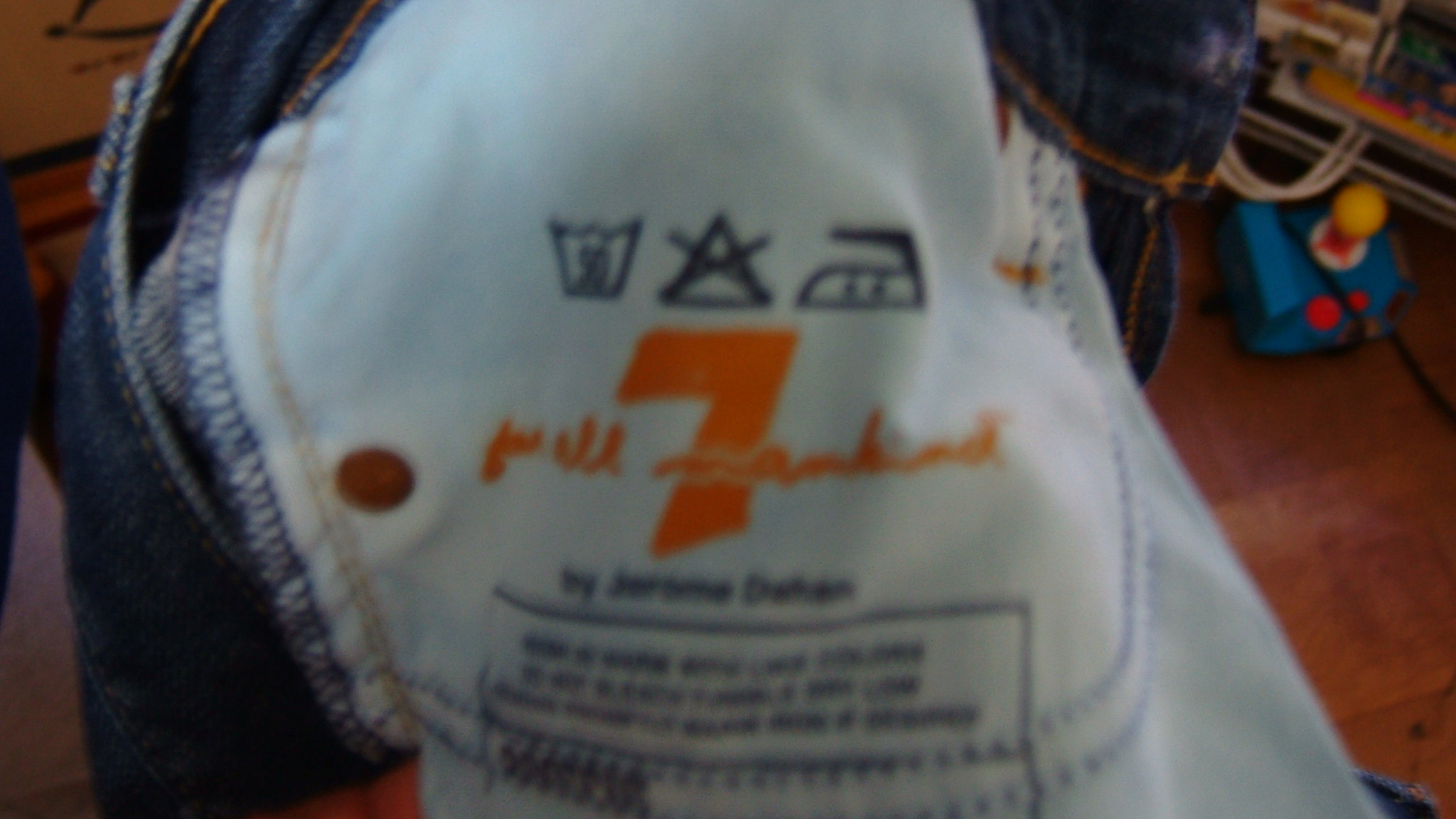This photograph depicts the inside of a pocket from a pair of blue denim jeans, turned inside out to reveal the white cotton label. The label prominently features an orange number 7, accompanied by script text that reads "for all mankind," though slightly blurry. There are six symbols indicating washing instructions, including a crossed-out bleach symbol. Below the orange number is a paragraph of text too blurry to decipher. The label is surrounded by the heavy blue denim of the jeans, featuring gold stitching, and there's a round metal disc, possibly a brad, near the edge of the white fabric. The background of the image shows a shiny mahogany wood floor with what appears to be a toddler's pull toy visible.